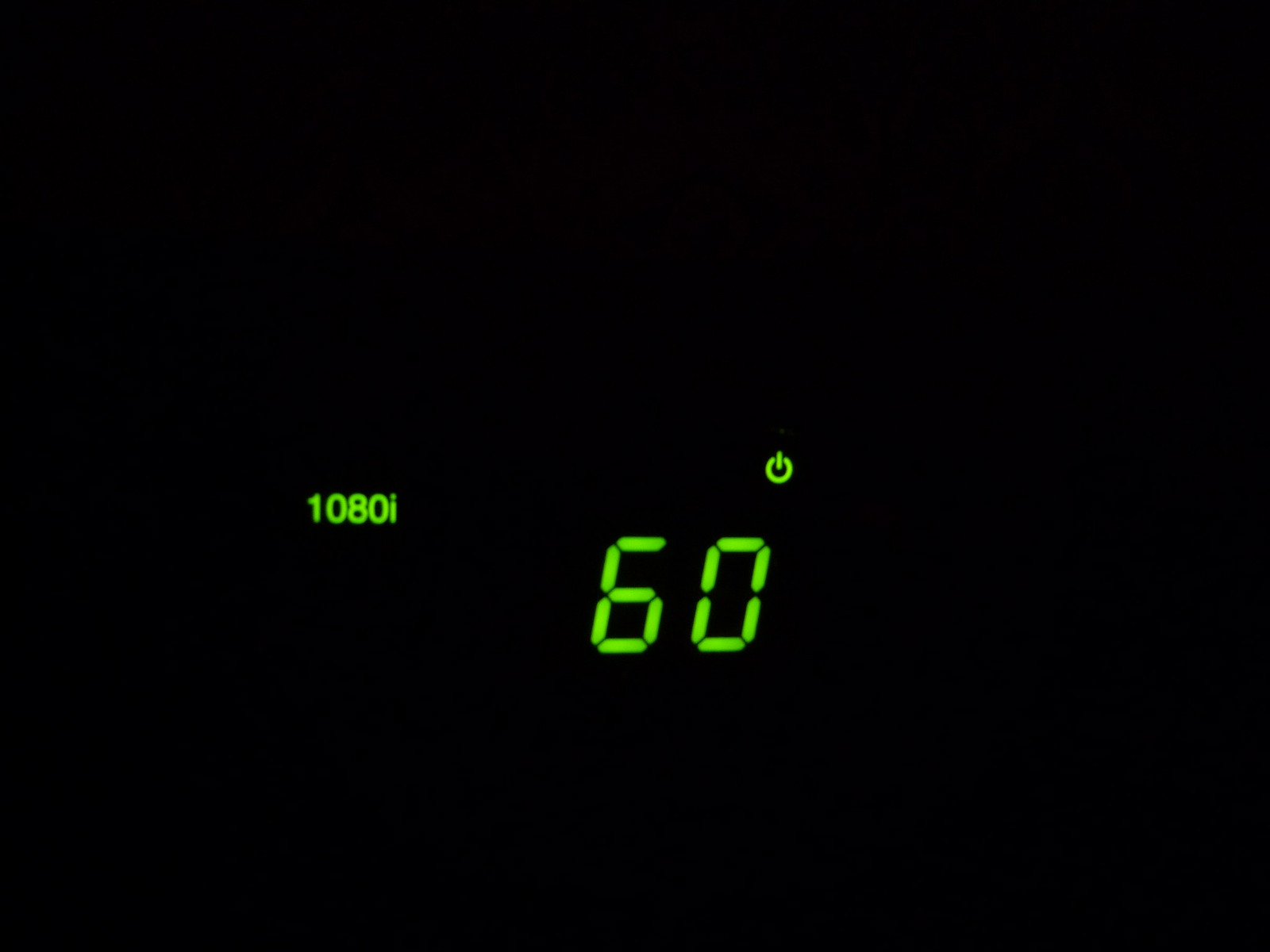This image showcases a digital display set against a completely black background, emphasizing its electronic nature. The screen features several distinct elements: at the upper center right, there is a universally recognized power on/off symbol, a circle bisected by a vertical line, indicating an interactive touch area for power control. Dominating the center left is the notation "1080i," a clear reference to a video resolution standard. Centrally positioned on the screen is the number "60," although its exact significance remains ambiguous - it could pertain to the frame rate (60 fps) typically associated with video recording, a temperature reading, or even a time duration. The green backlit numerical and symbolic readouts starkly contrast with the black background, reinforcing the screen's probable use in video or electronic settings, possibly on a tablet or similar device focused on displaying and managing video content.